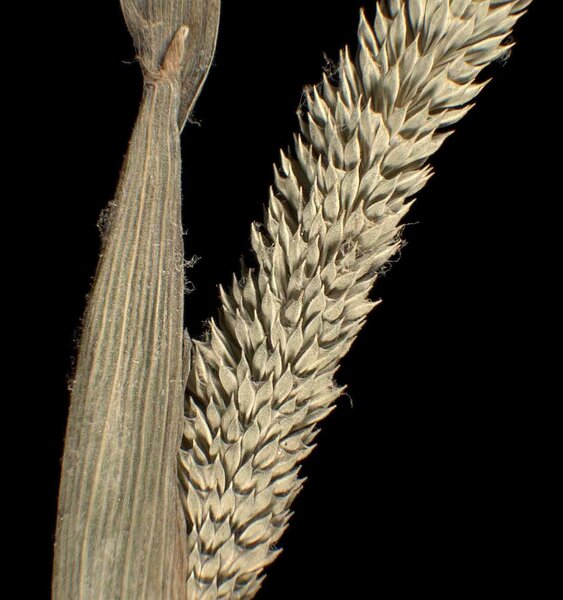The image captures a highly detailed, close-up view of a plant set against a pure black background, emphasizing the intricate features of the plant. On the left side of the image, there is an elongated, greenish-brown husk that strongly resembles that of a corn stalk, characterized by lighter vertical stripes and a pointed, twisted top that widens towards the bottom. The right side of the image shows a cluster of overlapping seed pods or mini leaves, extending diagonally from the bottom left to the top right corner. The seed pods are layered and display light green shades with hints of brown, adding texture. Both parts of the plant are delicately covered with fine dust or spider webbing, enhancing the natural, organic feel of the composition. The photograph is presented in a portrait orientation and leans towards a style of photographic representational realism, capturing the raw and unembellished beauty of nature.